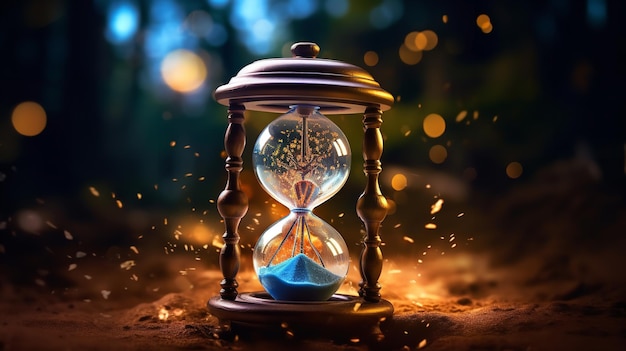This image captures an hourglass set within a meticulously carved wooden frame, defined by two ornate posts connecting a round wooden top and base. The hourglass itself has a classic figure-eight shape, with the top portion containing some golden specks and the bottom half filled with light blue sand that forms an elevated mound, almost reaching halfway up. The background features a mix of dark shades and blurred lights, creating an ethereal bokeh effect with glowing blue and orange dots scattered around. The hourglass is set on a ground that appears to be composed of brown dirt and wood chips, suggesting an outdoor forest setting. Additional light sources from various angles—behind, and to the right and left—emphasize the floating particles of sawdust, enhancing the mystical ambiance.